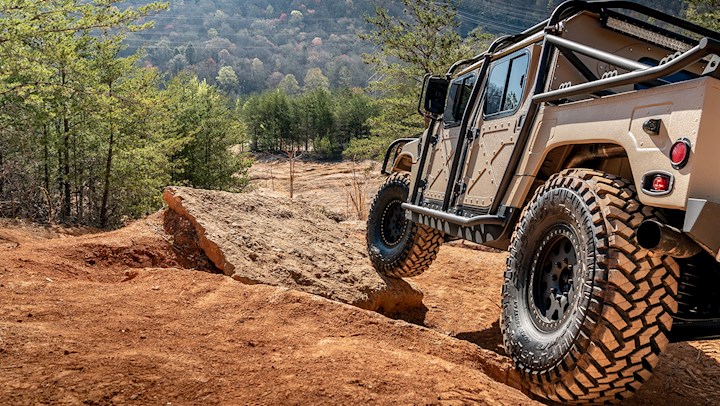The image captures a light beige, four-door Jeep-type all-terrain vehicle with a spacious open back and large, rugged tires caked with reddish-orange dirt. The vehicle, appearing robust and handsome, is navigating a rough, uneven dirt road lined with obstacles, including rocky terrain and a significant hole. The Jeep's front tires are perched precariously on the edge of a prominent square block of stone, creating a striking dynamic as it appears poised to leap off. The background reveals a landscape rich with trees and dominated by a hillside or mountain, enhancing the adventurous atmosphere. The photograph's clarity and composition effectively convey the rugged beauty of the scene, filled with natural elements and the challenging terrain, highlighting the vehicle's capability and robust design.